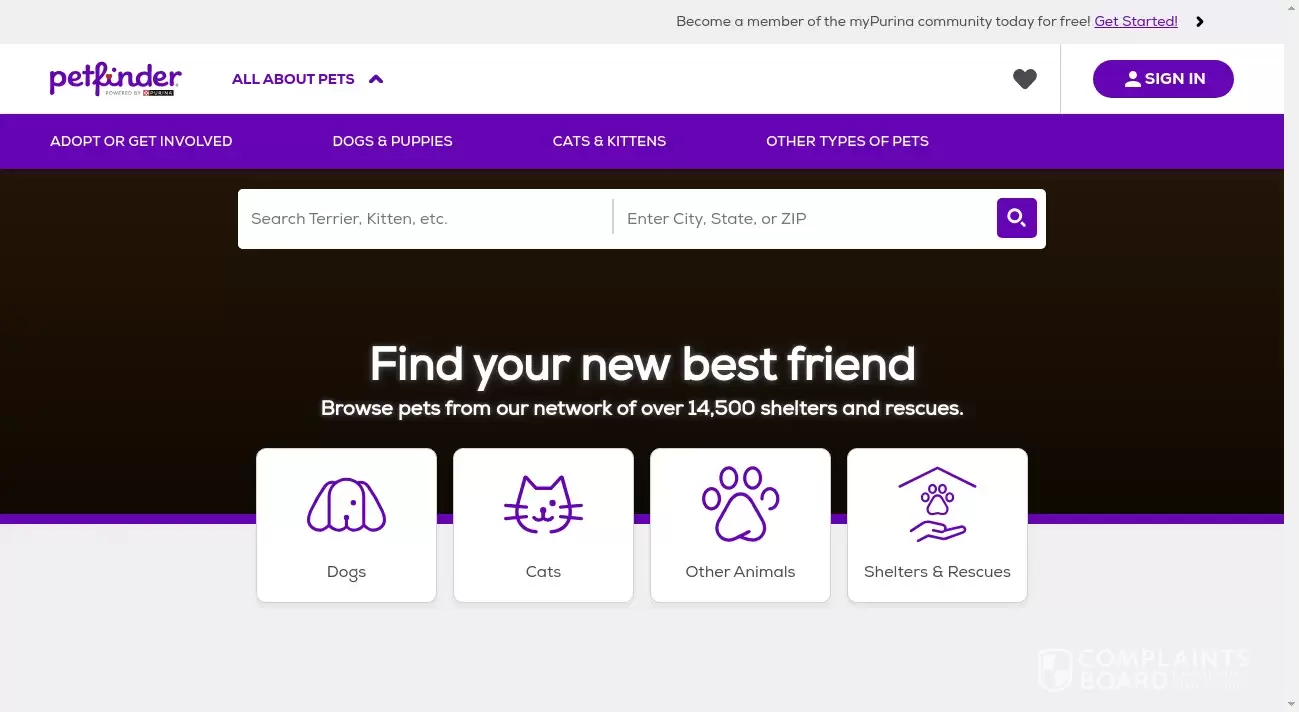This is a detailed screenshot of the Pet Finder website, showcasing its user-friendly interface and extensive features designed to help you find and adopt pets. The Pet Finder logo is prominently displayed in purple, accompanied by the tagline "Powered by Purina." At the top, a vibrant banner invites users to "Become a member of my Purina community today for free," with a prominent purple "Get Started" button.

The site includes various sections to streamline navigation: "Adopt or Get Involved," "Dogs and Puppies," "Cats and Kittens," and "Other Types of Pets." A Sign Up or Log In button is available for easy access to personalized features.

A central search bar encourages users to find pets by entering terms like "Terrier" or "Kitten," along with their city, state, or zip code. Just below, white text on a dark background reads, "Find your next best friend. Browse pets from our network of over 14,500 shelters and rescues."

The homepage features distinct sections for different animal categories: 
- A "Dogs" section highlighted by a purple dog face icon.
- A "Cats" section symbolized by a purple outline drawing of a cat.
- An "Other Animals" section represented with a paw icon.
- A "Shelters and Rescues" section marked by a paw with a hand underneath it, both icons also in purple.

The layout combines a clean, white color scheme at the top and bottom with a dark black section in the middle, accentuated by a blue or purple bar above it, creating a visually appealing and organized homepage.